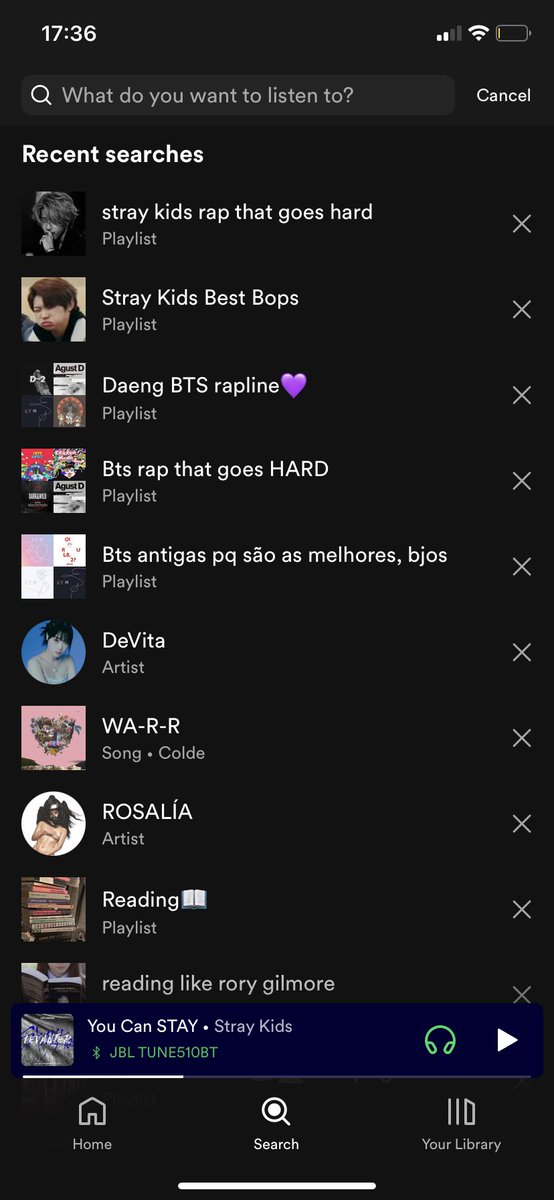The image displays the screen of a phone running the Spotify app, set in dark mode with a predominantly black background. At the top of the interface, a search bar poses the question, "What do you want to listen to?" beneath which recent search history is displayed. The visible searches include curated playlists and artists related to K-pop and rap. The top search result reads, "Stray Kids rap that goes hard," followed by additional playlists such as "Stray Kids best bops" and "Dang BTS rap line, Purple Hearts playlist." The sequence continues with "BTS rap that goes hard," "BTS, Antigas, P.K.," and then the artist DeVita, noted by a capitalized "V." There's a song titled "WA-R-R" by an artist named Coldy, a mention of the artist Rosalia, and playlists like "Reading" and "Reading like Rory Gilmore." A song currently playing, identifiable by its title presented at the bottom of the screen, is "You Can't STAY" by Stray Kids, with "STAY" emphatically capitalized.